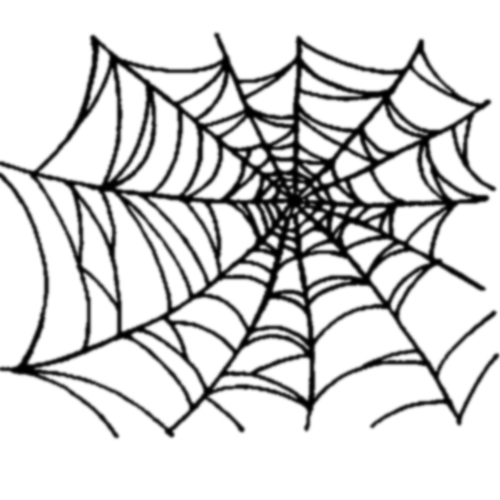This image showcases an intricate, black spiderweb drawn on a plain white background. The web, illustrated with simple black ink, displays a geometric and somewhat spiky appearance, with its structure becoming more compact toward the center. The design features multiple layers, each radiating outward and creating a target-like focal point. The spiderweb's outer layers gradually expand, showcasing curved patterns typical of such webs, with around ten distinct sides that repetitively extend outwards. The overall effect is a detailed, radiating geometric pattern that captures the essence of a spider's craftsmanship.